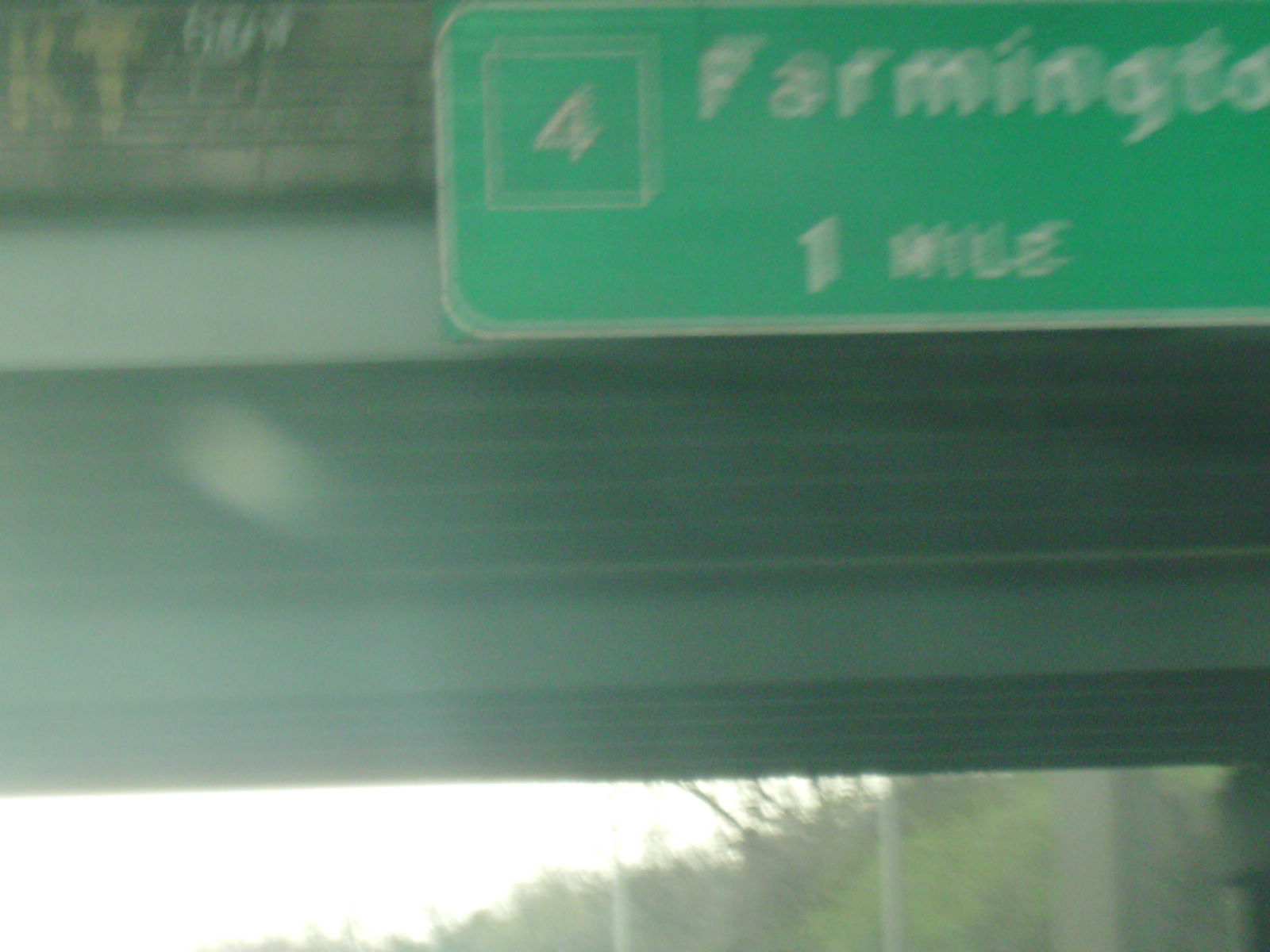This image, though of low quality, captures a moment from a moving vehicle on a major roadway. The blurry and overexposed photograph presents a challenge in clarity, yet certain details remain discernible. It depicts a green sign affixed to an overpass or bridge, viewed from the ground up. The sign prominently displays the number "4" within a box, accompanied by the partially obstructed text, "Farmington," where the 'N' in 'Farmington' is notably cut off. Additionally, the sign indicates that the destination is "one mile" away. To the left of the main sign, there is additional, indecipherable text. The overall washed-out effect adds a sense of motion and urgency to the scene.